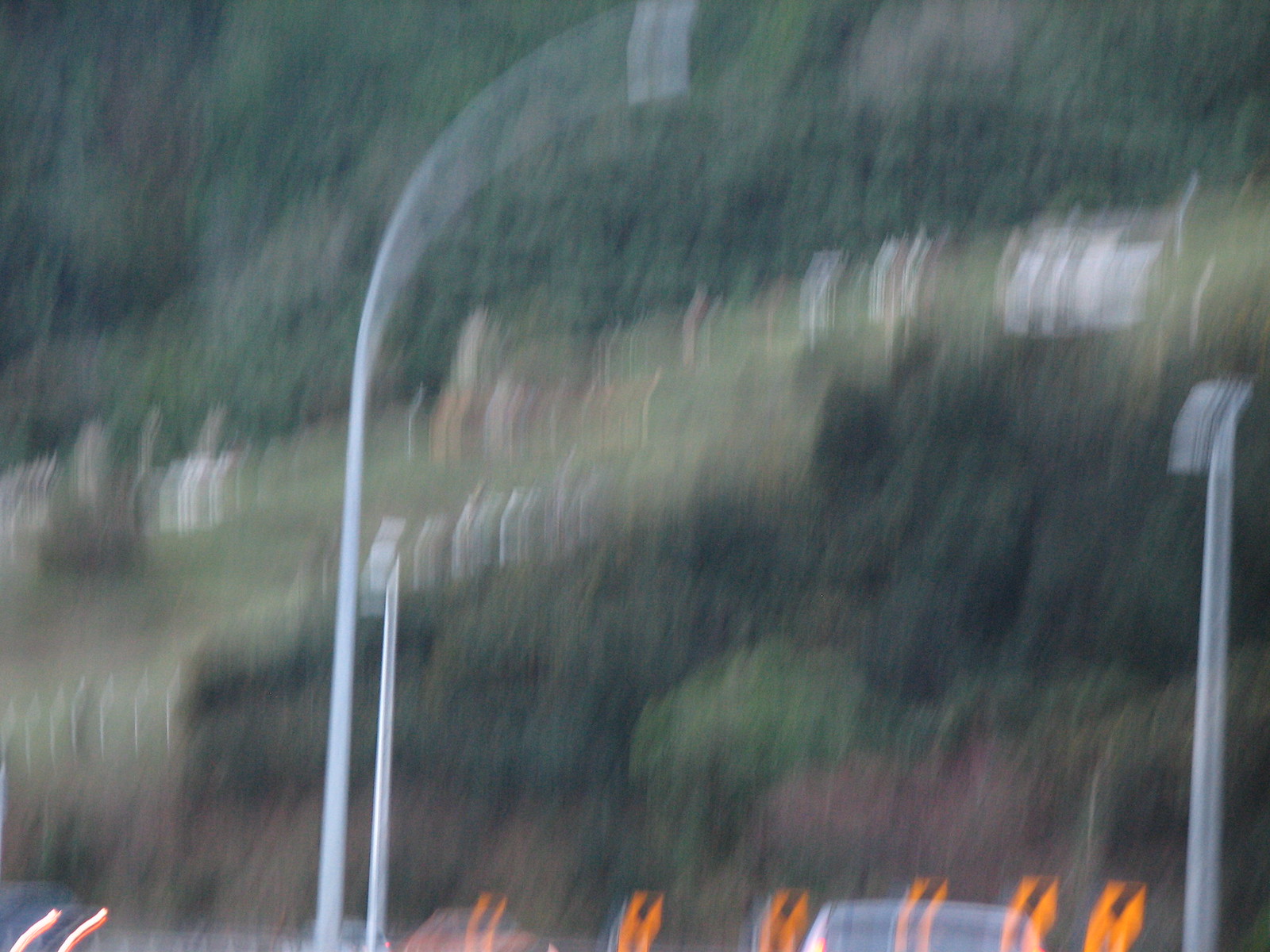A blurry image depicts the side of a mountain featuring distinct layers of flora and rock formations. The mountain presents several levels, showcasing a mix of trees, rocky outcrops, and patches of greenery that are not trees. There are large street lamps mounted on tall silver poles, indicating this could be a rest area. In the vicinity at the same level as the camera, a few cars can be seen, including a white and a red one, parked in what appears to be a parking lot. Additionally, there's a section that seems to be covered with grass, suggesting the presence of a rest stop or viewing area. Despite the blurriness, one can infer that the area may also include a bridge, adding to the complexity of the scene. The image captures the interplay between natural and man-made elements, albeit in a very unclear manner.